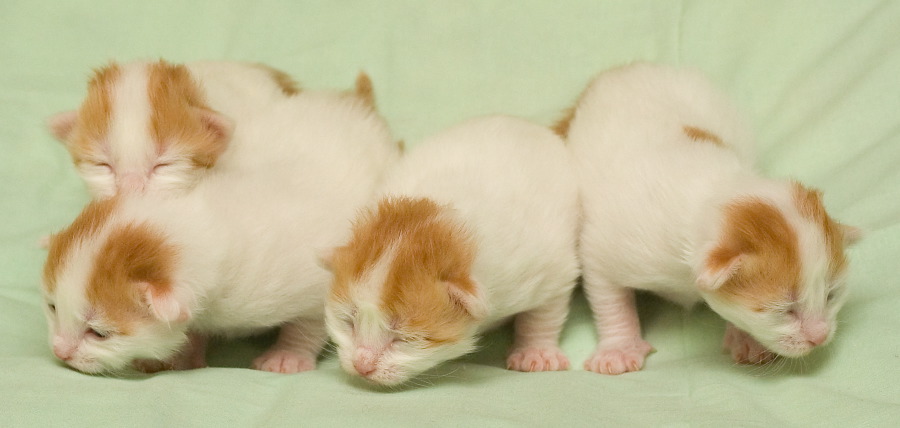This vibrant, color photograph captures the pure cuteness of four newborn kittens nestled closely together on a light green blanket. Each kitten, still unable to fully open their eyes, is adorned with predominantly white fur, accentuated by patches of light brown fur around their ears, giving the illusion of tiny white mohawks. The soft pinkness of their noses and paws highlights their tender age. Arranged in a tight cluster, the kittens are positioned in various angles – the one in the top left has its eyes tightly shut, while the one at the bottom left seems to have its eyes slightly open. The delicate and intimate setting on the soft surface amplifies their vulnerability and the overwhelming cuteness of these incredibly soft, young creatures.